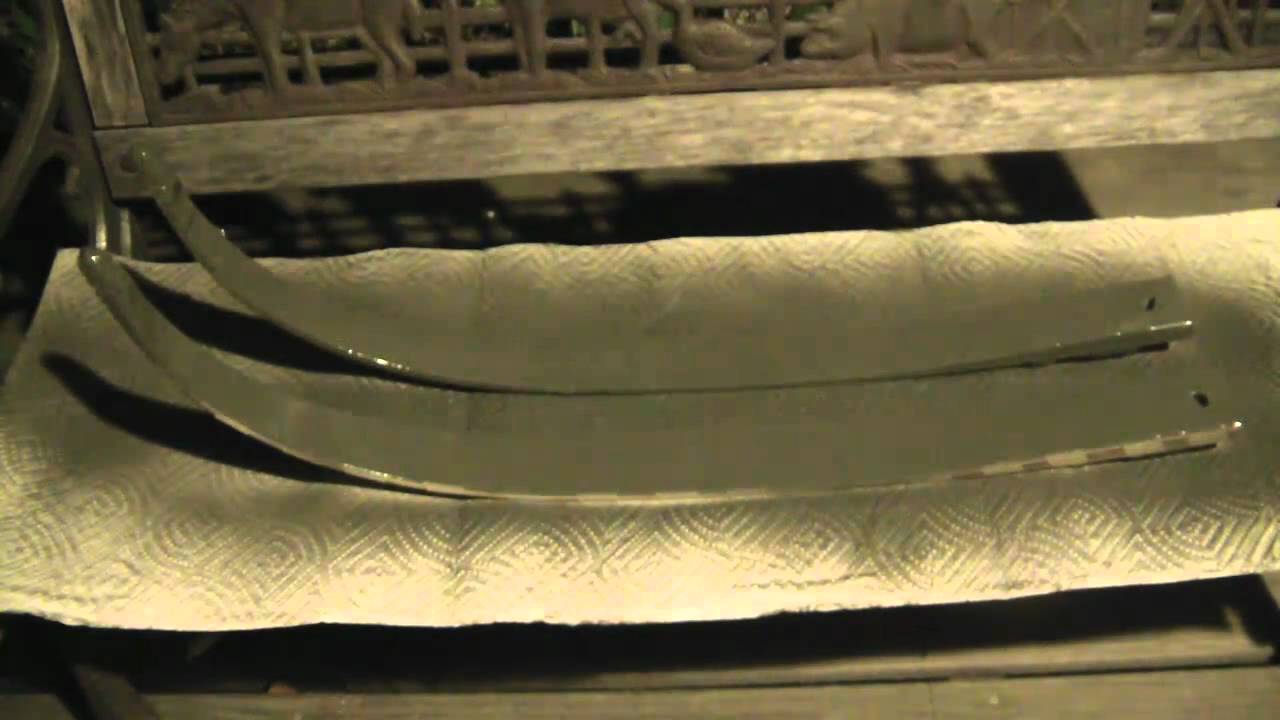This is a close-up photograph of two long, aged metal objects with a dull brass coloration, lying horizontally on a similarly colored, textured fabric. The objects, both made of metal, curve gently upwards toward the left to a rounded point, while the right ends feature small drilled holes. They are set against a fabric backdrop with intricate, embroidered diamond patterns blending in with the fabric's color. The photograph also captures compression artifacts indicative of low-quality digital imaging, adding a blurry effect to the scene. In the distant background, part of a bench's metal backrest is visible, providing context to the setup.